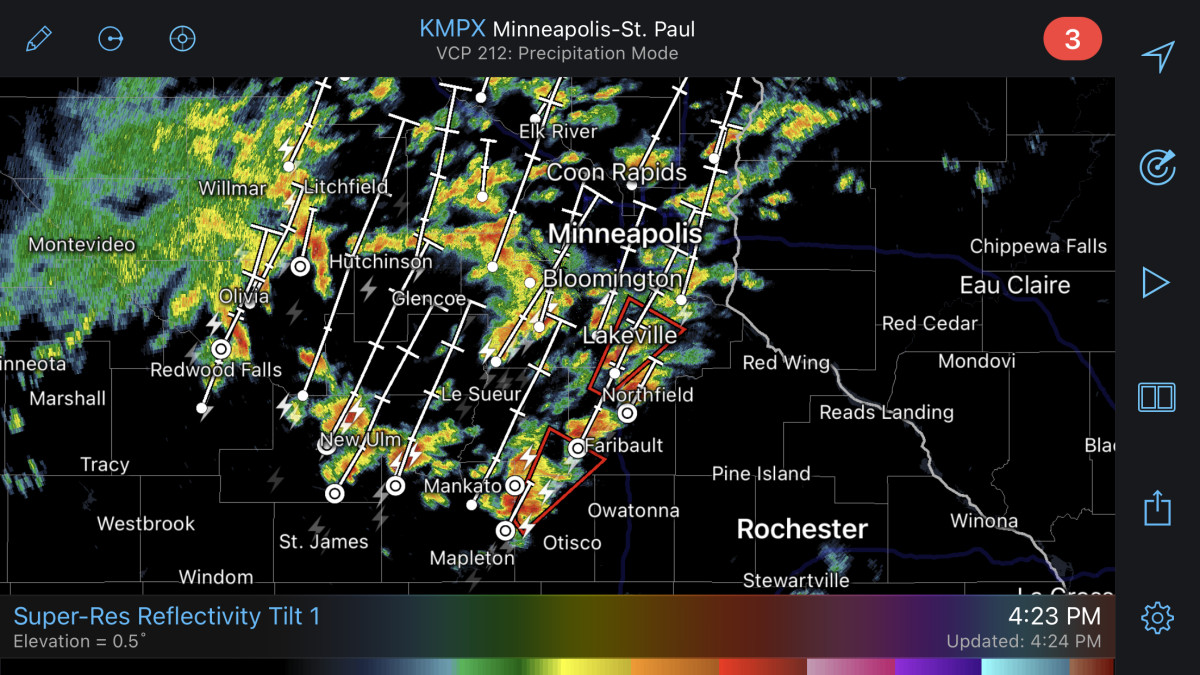A detailed weather map centered on the Minneapolis-St. Paul region, clearly marked at the top in white text. The map is provided by KMPX, as indicated on the left side of the title. Below the title, the mode is set to VCP-212 Precipitation Mode, with a prominent red circle containing the number three to the right.

The map itself is vividly color-coded, displaying a mixture of green, yellow, and bright orange areas, indicating varying levels of precipitation intensity, with the brighter colors representing more severe weather conditions. Minneapolis is centrally located and marked in white text. Below, other key locations such as Bloomington, Lakeville, Red Wing, Reeds Landing, and Winona are noted, aligned along a long white line extending towards the right.

Additionally, Rochester is clearly marked in bold white text to the left of this line, while Chippewa Falls is situated in the upper-right portion of the map, just above EAU CLAIRE. In the bottom-left corner, the map provides technical details: "Super Res Reflectivity Tilt 1" in blue text, along with "Elevation = 0.5."

A gradient color bar at the bottom of the map ranges from gray to deep colors like green, yellow, orange, red, pink, purple, light blue, and finally ends in orange, which corresponds to the precipitation levels on the map. This section is accompanied by an update timestamp of 4:24 PM.